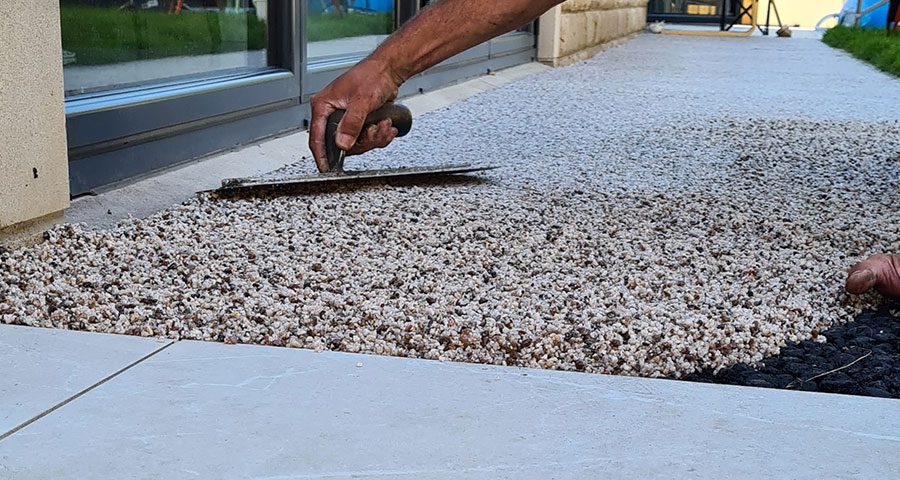In this ground-level photograph, we see a Caucasian man meticulously working on a textured walkway. He is using a leveling tool with a dark brown wooden handle and a smooth metal bottom to evenly distribute a rough, variegated cement mixture, which includes white, brown, and gray pebbles. The walkway, composed of many small stones, is being laid behind a gray sidewalk that spans the bottom of the image from left to right. The area features contrasting black stones in the lower right corner, with a blend of pebbles making up the rest of the surface. The man's right hand, tanned from the sun, firmly grasps the tool, while the thumb of his left hand is visible on the right edge of the frame, aiding his balance. In the background, to the left side of the photo, there is a building with tan-colored stones and bricks, and several windows with black trim on the bottom. A sliding glass patio door with a metal frame is also visible, suggesting this construction is taking place outside a house with dirty white plaster bricks. The upper right corner shows a patch of grass adjoining the newly poured cement, adding a touch of greenery to the scene.